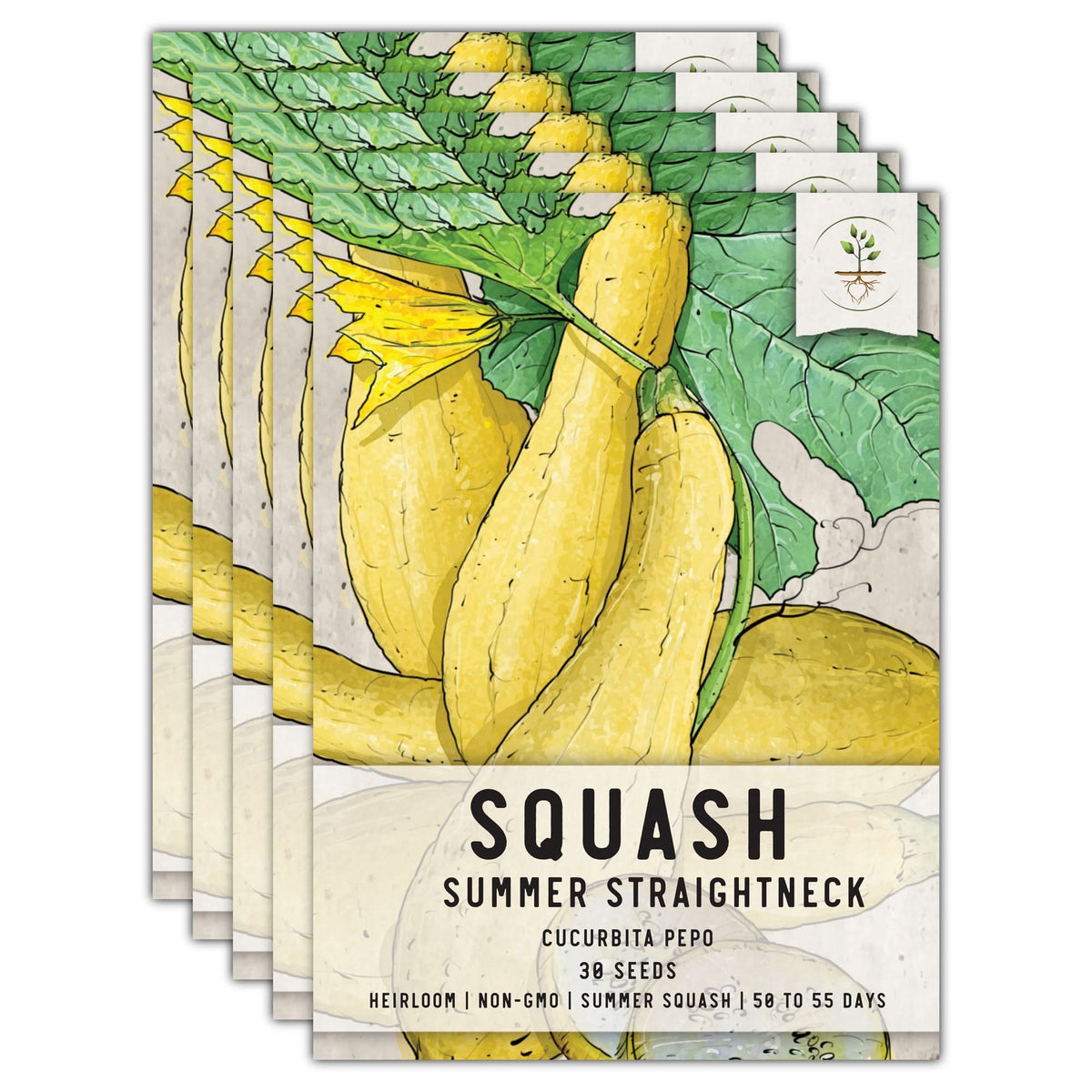The image showcases a detailed, hand-drawn illustration of yellow squash, specifically focusing on packets of "Summer Squash - Straight Neck" seeds. These heirloom, non-GMO seeds come in packets, each containing 30 seeds and promising a growth period of 50 to 55 days.

The drawing prominently features two vertical squashes lying side by side, with another horizontal squash behind them. In the background to the left, a fourth squash is visible, also positioned vertically. The upper left corner of the image is adorned with green leaves and a bright yellow squash flower, adding a touch of natural vibrancy.

There are a total of five packets stacked on top of each other, clearly displaying the label that reads: "Squash Summer - Straight Neck, 30 seeds, Heirloom, Non-GMO Summer Squash, 50 to 55 days." The overall presentation is both informative and visually appealing, capturing the essence of these summer squash seed packets.